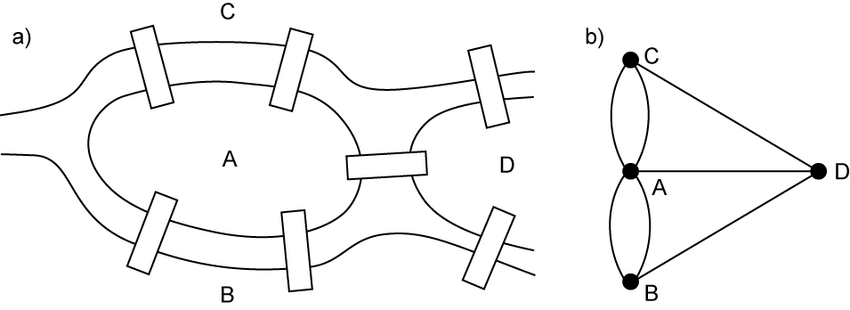This image is a black-and-white diagram consisting of two main parts, labeled A and B. 

On the left, labeled as 'A', there is a diagram that resembles a series of interconnected ovals or eyeglasses with braces. The image displays one and a half ovals, with the oval on the left divided into four sections marked A, B, C, and D. Each section connects through small white rectangles: four on the left oval, one near where the nose would go if it were glasses, and two on the right half of the oval. The diagram creates a looping structure with the labels arranged such that A is inside the left loop, C is above, and B is below. The oval partially shown on the right features a label D at the connecting part.

On the right side, labeled 'B', the diagram depicts two horizontally-aligned conical shapes positioned end-to-end. The top cone is labeled C, the bottom B, and the middle section where they meet is labeled A. Additionally, there's a connecting point marked D at the intersection of the cones. This side also displays lines forming triangular shapes extending from the tips of the cones, enhancing the conical representation.

Overall, the image juxtaposes two different diagrammatic structures, one resembling a chain of ovals with labeled segments and connecting braces, and the other depicting intersecting cones with labeled vertices and base intersections.